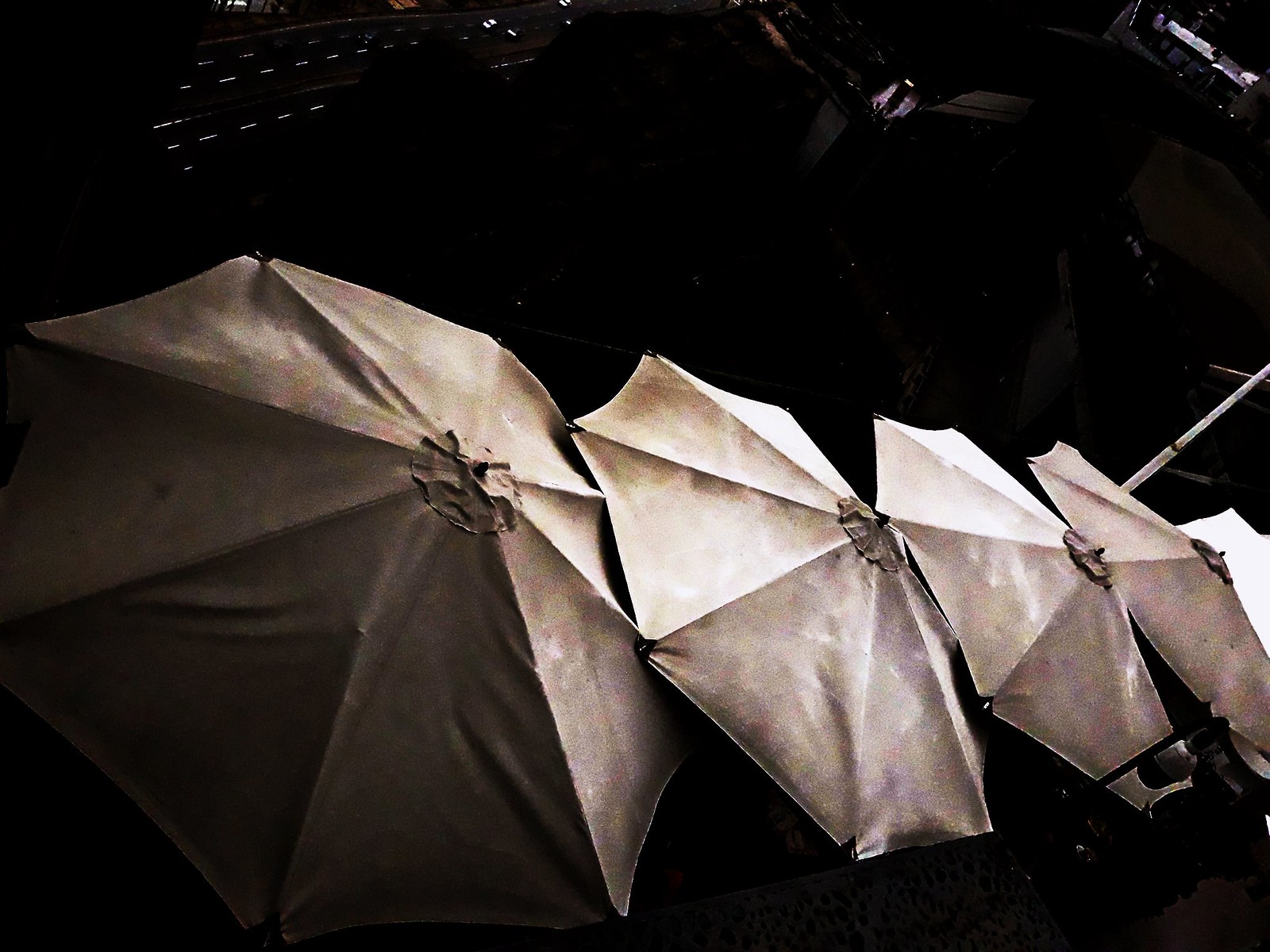The image depicts a nighttime scene featuring an arrangement of five large, gray patio umbrellas, possibly located in an outdoor dining area. All the umbrellas are open and oriented upwards, overlapping each other as they extend from the left side of the image to the right. The background is predominantly black and indistinct, with some light slits visible towards the top left, suggesting minimal lighting, possibly from distant sources or reflections. A small peg shape protrudes upwards towards the top of the image, while a segmented pole is visible on the right side, extending over the umbrellas. The fabric of the umbrellas appears to be gray, with some white reflections indicating the light source. The overall perspective and lighting give the scene a slightly confusing and surreal quality.